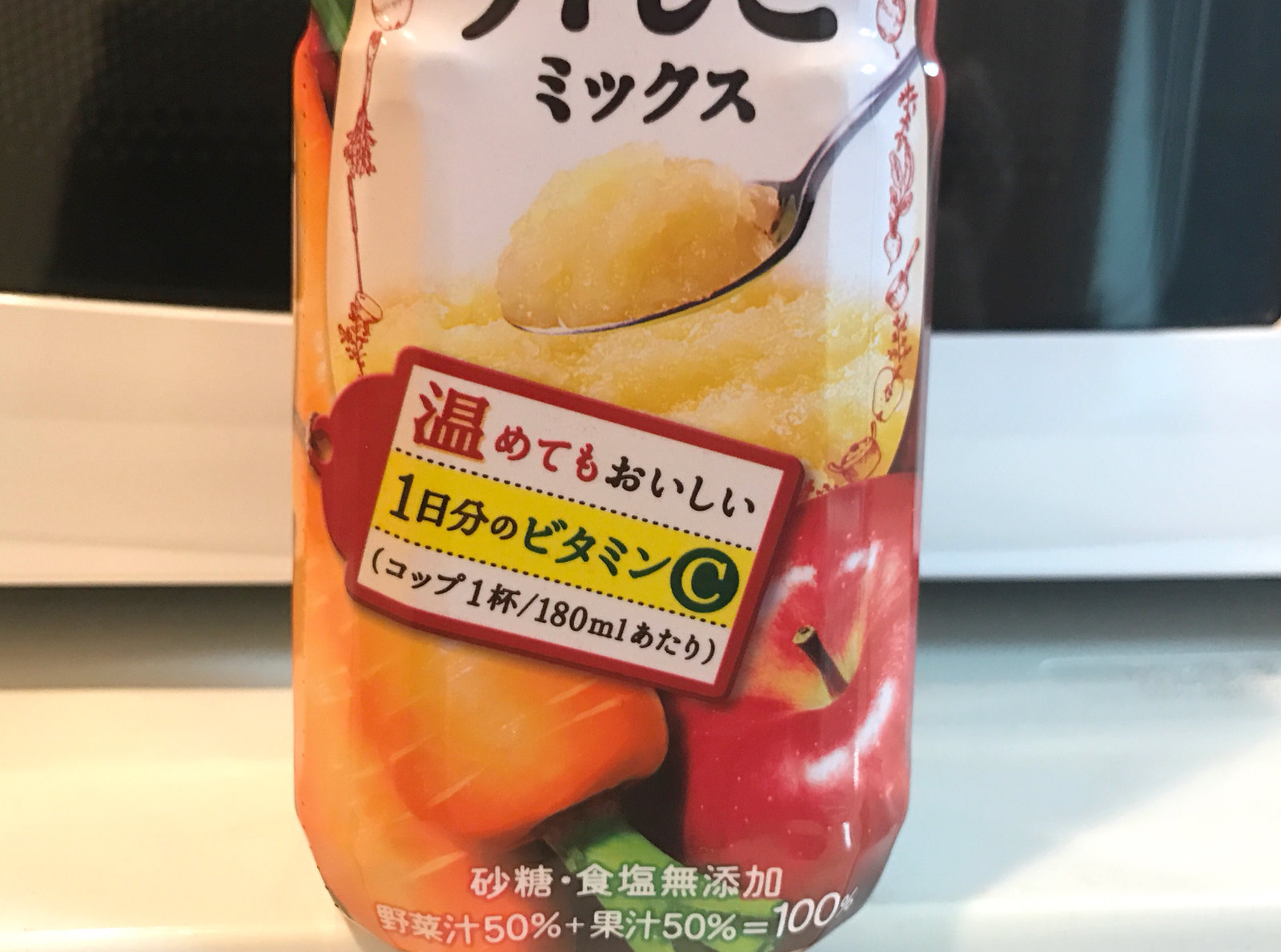This color photograph features a food container adorned with Japanese kanji text, making the exact contents unclear. The container's label displays black and red Japanese characters, and includes a distinct yellow band with additional black writing. Prominently visible is a spoon holding a rich, yellow sauce that resembles applesauce. Below this image, the label showcases vibrant pictures of two orange carrots with green stems and a red apple. The container indicates a volume of 180 milliliters and features a mathematical expression "50% + 50% = 100%" interspersed with Japanese characters. The photo is set against a black and white background with the container resting on a white tabletop.